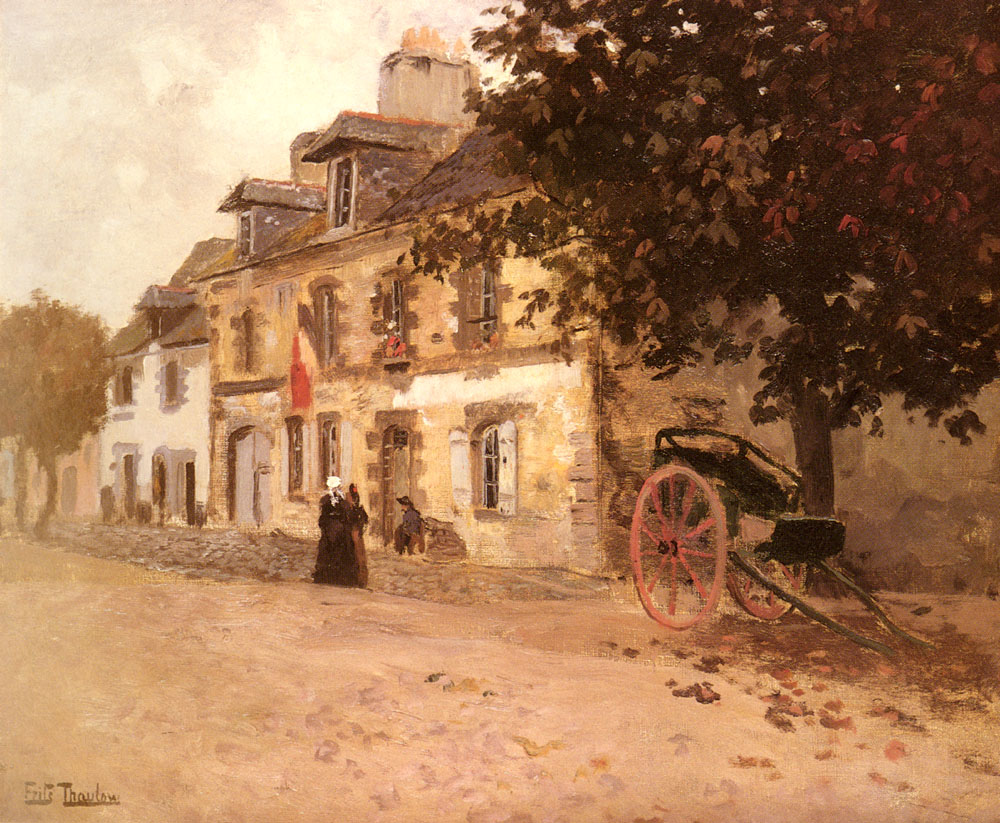This detailed oil painting titled "A Village Street in France" by artist Frits Thaulow, created in the late 1800s around 1906, captures a picturesque scene of a two-story stone building in a rural setting. The building, with its brown stone finish and keystones around the front door and windows, features four windows on the upper level and four on the lower level. The structure appears to widen towards the viewer and tapers off to the left, with a noticeable tower visible in the distance. The roof includes two dormers, adding to the architectural charm.

On either side of the building, lush trees frame the scene; one particularly large tree, with red and brown leaves, occupies the right side, partially shading a horseless carriage. The red-wheeled buggy sits at the base of the tree, its shaft resting on the dirt-covered ground, reminiscent of a slower-paced era. 

In front of the building, on a dirt to cobblestone path, stand two women dressed in long 19th-century attire. One wears a white bonnet, the other a red headdress. A dog stands attentively at the front door, enhancing the homely feel of the scene. Additionally, it appears there is a third woman seated by the front entrance, adding to the narrative depth of the painting.

The artist’s signature can be found in the lower left corner, though it’s quite small and reads "Fritz Truslow." This genre painting with an impressionist style wonderfully encapsulates the serene yet vibrant village life of early 19th-century France.